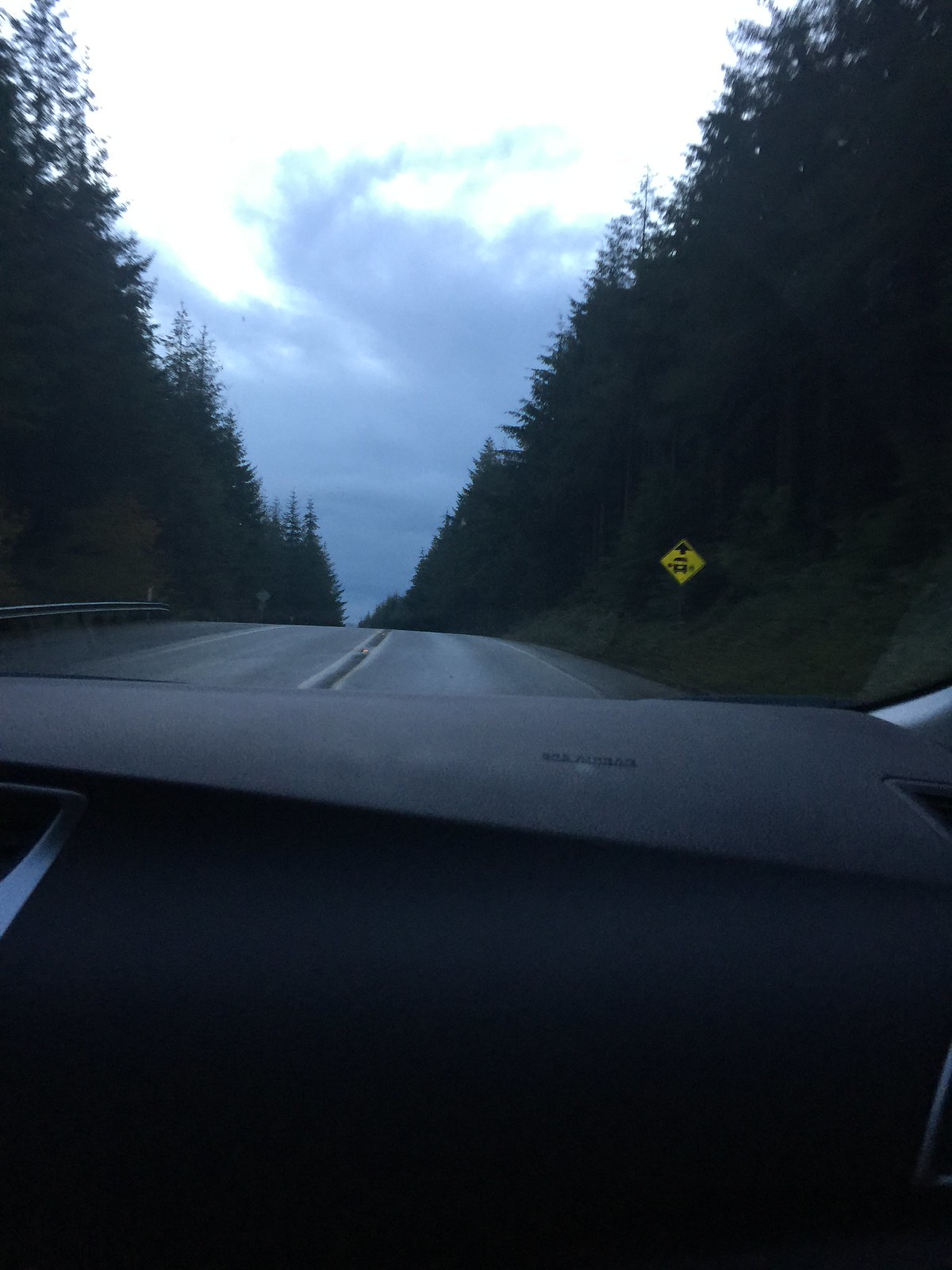A scenic road stretches into the distance, framed by dense clusters of trees on both the left and right sides of the image. The sky above is predominantly bright white, punctuated by ominous dark clouds that hint at an impending storm. In the center, white road signs with text point upward, providing directional information. Below, the black asphalt road features a distinct yellow line dividing the lanes. The photo is taken from within a vehicle, capturing the gray plastic dashboard and offering a view through the windshield, giving a sense of a journey underway.